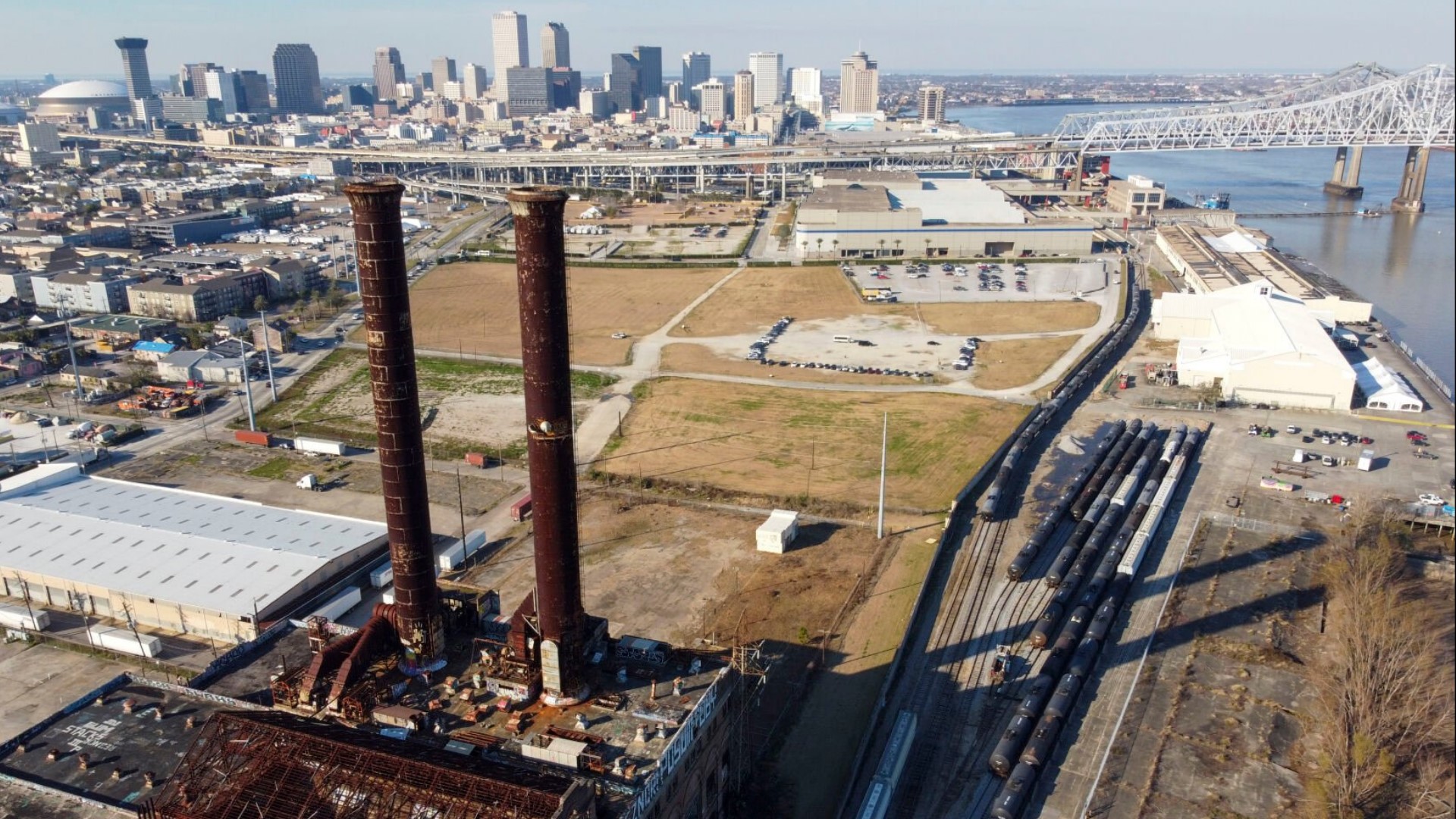This aerial photo captures a bustling cityscape with a multitude of details. In the foreground, the image is taken from atop a building looking downward. The city is dotted with various structures, including numerous industrial facilities, as evidenced by the large, rusty smokestacks located prominently in the left corner. Near these stacks, there's a significant white building and several empty plots of land with patches of dead grass. On the right side of the photo, a line of burned-out trees stands near what seems to be either trucks or trains, likely part of a train yard or industrial transport system.

Further into the city, a river with a bridge spanning across it is visible, accompanied by a concrete shoreline. There's a prominent large white building along this shoreline. Moving beyond the foreground, the photo reveals residential areas with houses and apartment complexes interspersed with roads and railroad tracks, illustrating the city's intricate web of infrastructure.

In the distance, the city's skyline boasts tall skyscrapers, signifying a vibrant metropolitan area. In the upper left quadrant, a stadium with a rounded, domed top can be seen, adding to the city's varied architecture. The sky is overcast, casting a dull hue over the scene, and the adjacent body of water, potentially a lake, mirrors the overcast environment with its muted colors. Overall, this East Coast-looking cityscape captures the blend of industrial might and urban living.